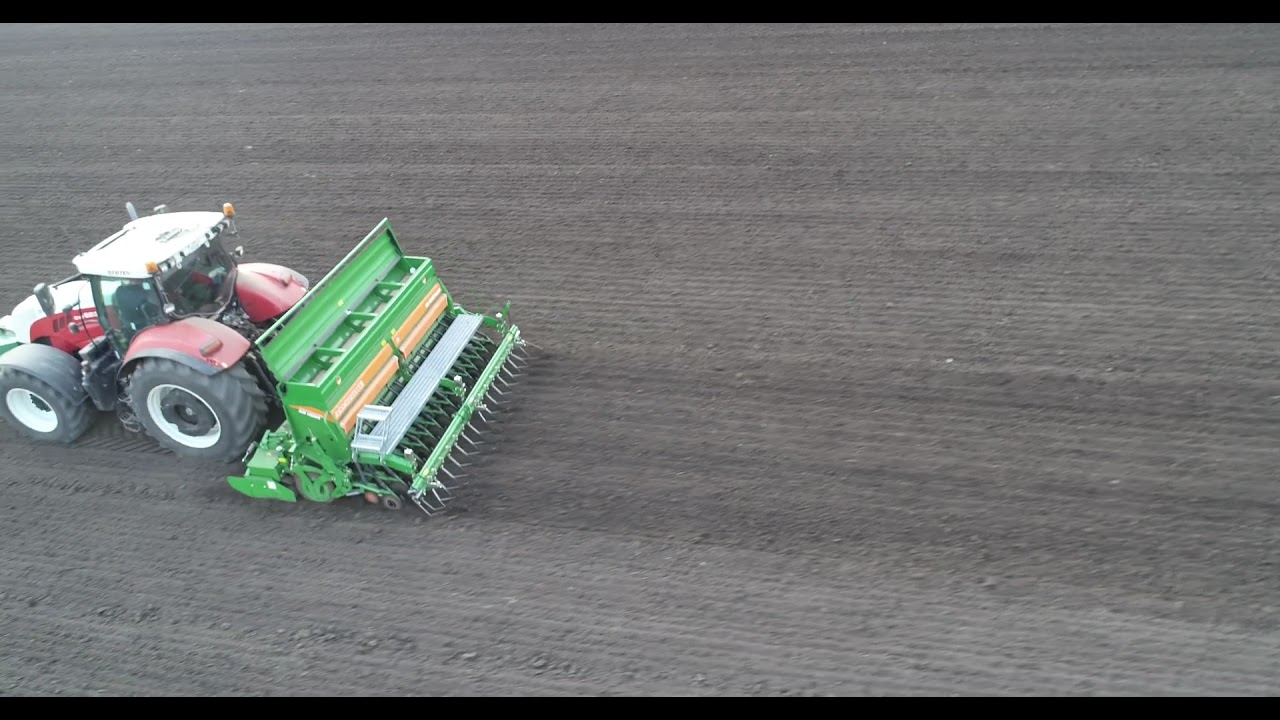This detailed aerial photograph, likely taken from a drone or crane, captures a vast brown farm field being meticulously plowed by a large red tractor. The tractor, visible towards the left of the image, features an enclosed cabin with a white roof, large black tires with white rims, and red paint on its body and wheel coverings. It is towing a green plowing machine equipped with silver metal rakes, which are creating the visible horizontal parallel lines in the soil as it moves across the field from left to right. The field shows clear striations both above and below the tractor, evidencing multiple passes over the area. The photograph is framed with thin black strips at the top and bottom, with no borders on the sides.